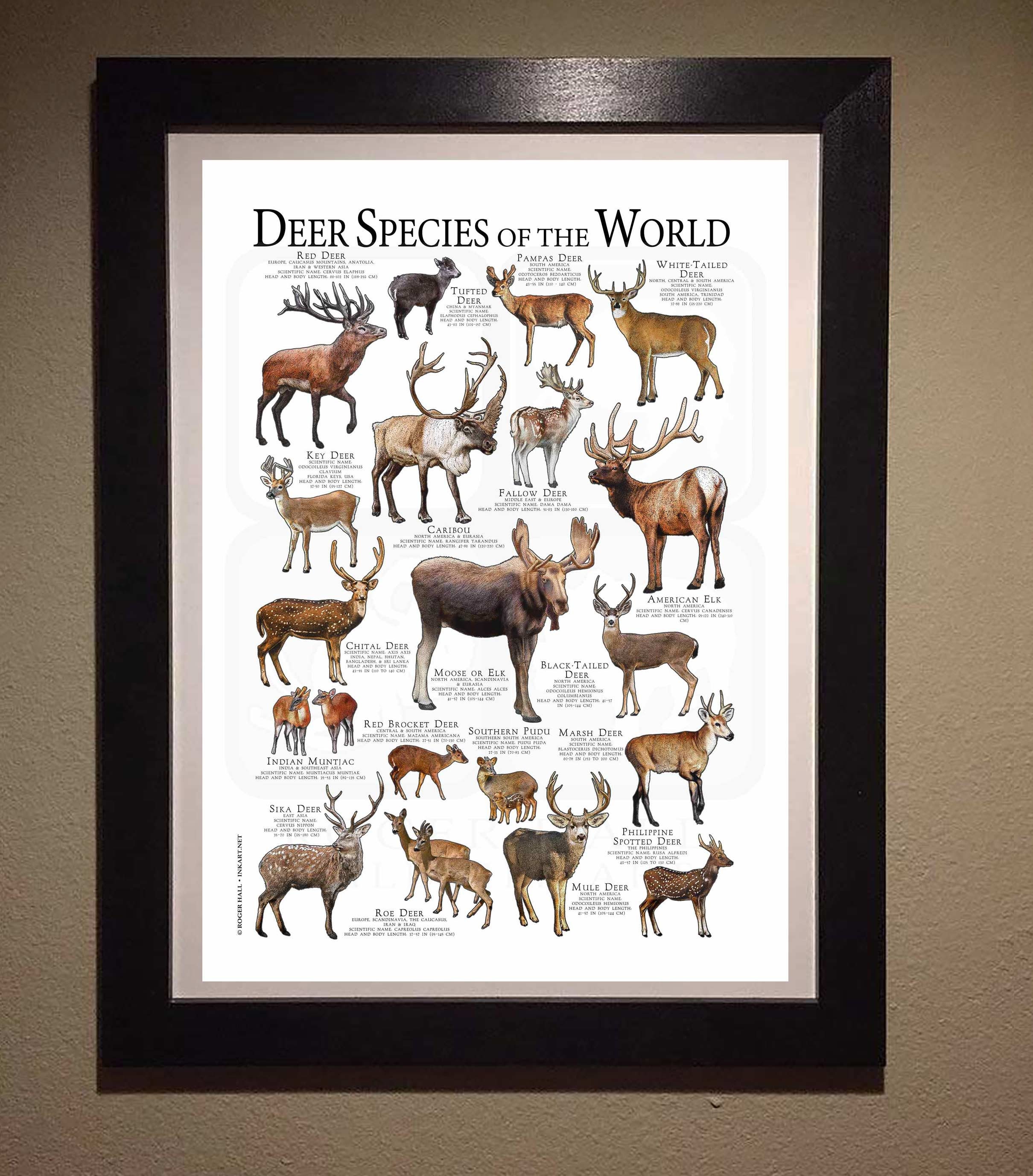The image depicts a detailed, full-color infographic titled "Deer Species of the World," framed in a plain black wooden frame and hung on a textured gray wall. The infographic features lifelike drawings of around two dozen different deer species, ranging in color from white to dark brown. Some deer have spots, others have antlers, and notable species include the red deer, white-tailed deer, and Philippine spotted deer. Each illustration is accompanied by a name and a small, unreadable descriptive paragraph. The infographic's presentation includes a gray mat with a white paper background, adding depth and contrast to the meticulously detailed display.